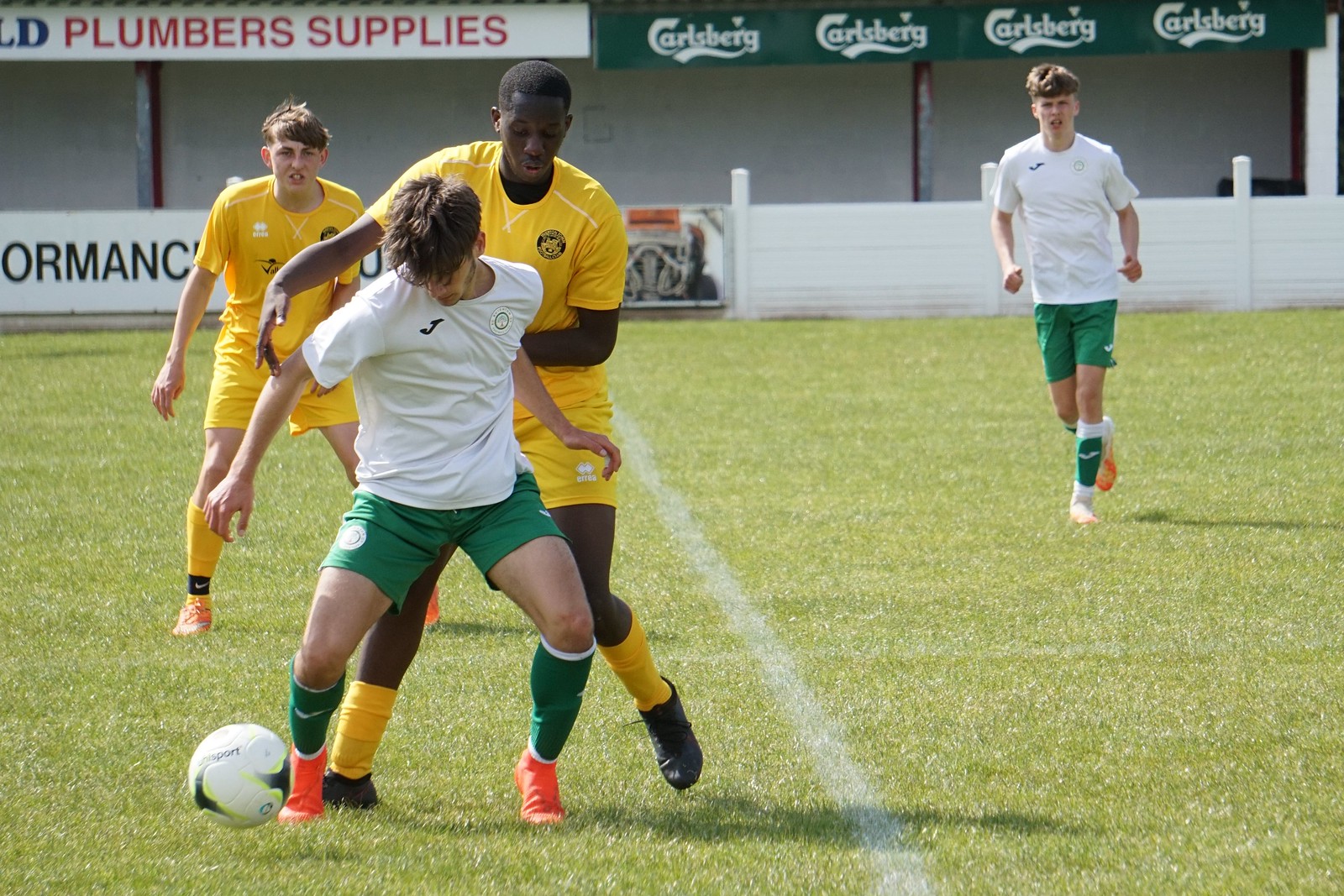This detailed photograph captures an intense soccer match taking place on a well-kept field. The focus is on four young men deeply engrossed in the game. Two players, one white and one black, are part of a team wearing yellow uniforms—yellow shirts, shorts, and black and yellow socks. The black player, a notably tall and imposing figure, is actively trying to dispossess the ball from a member of the opposing team. This opponent, dressed in a white shirt, green shorts, and matching white and green socks, is defending the ball determinedly. The scene is set against a backdrop of a stadium wall adorned with advertisements, including repeated signs for "Plumber Supplies" and "Carlsberg." The atmosphere suggests a serious, competitive nature to the match, indicating it could either be an amateur or professional level game.